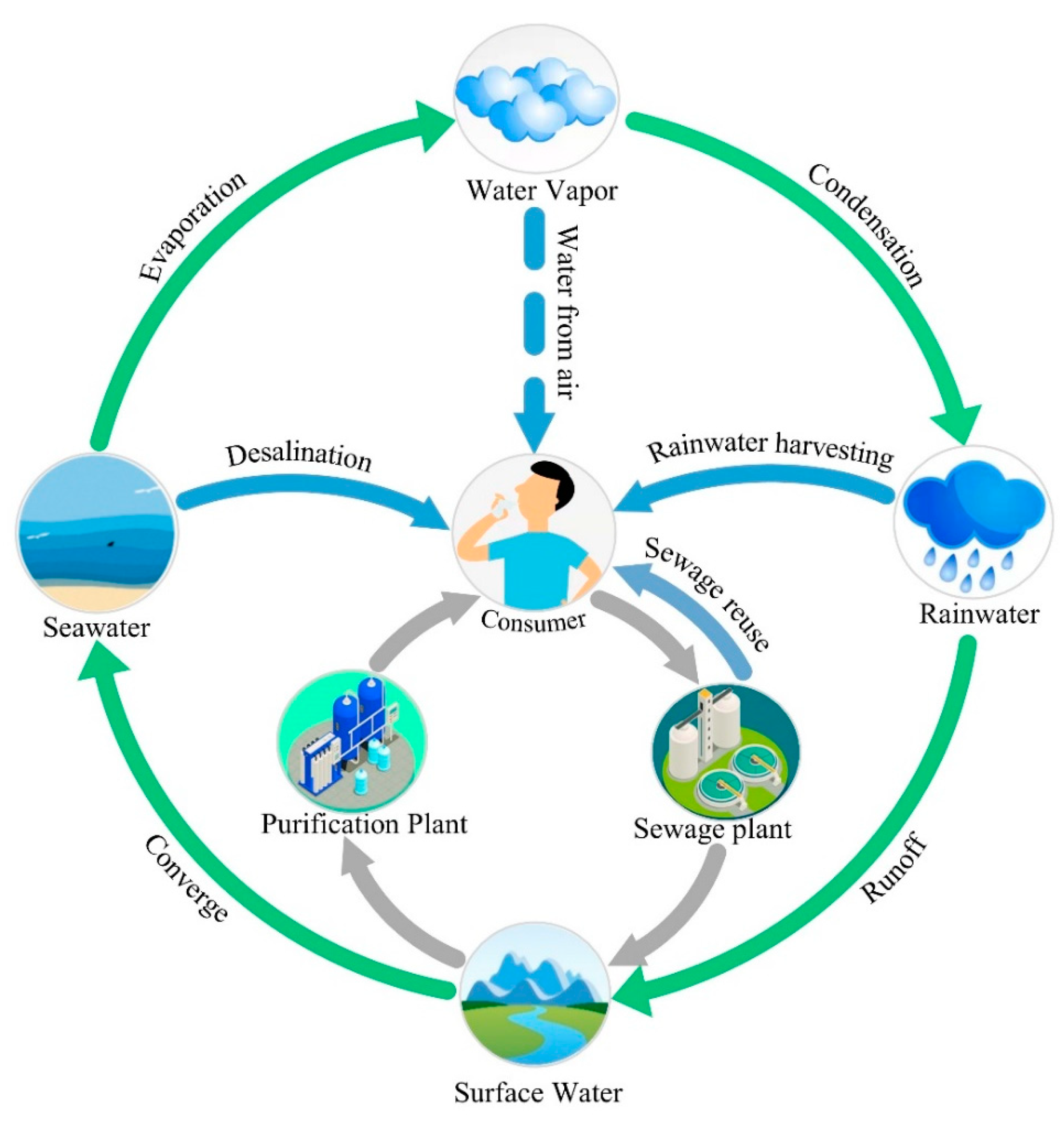The image depicts a detailed flowchart illustrating the water cycle with various stages and processes, emphasizing the journey of water and its interaction with the consumer. At the center, there is a circular symbol featuring a human figure with black hair, beige skin, and a blue shirt labeled "consumer." Several arrows radiate towards the consumer from different stages of the water cycle.

Starting at the top, there is a cloud symbol labelled "water vapor," with a green arrow indicating "condensation," transitioning to another symbol for "rainwater" depicted with droplets in shades of blue. This process leads to "runoff," symbolized by a green arrow directing to "surface water," an image representing rivers and glaciers. The flow continues with an arrow titled "converge," leading to a "seawater" symbol. From seawater, a green arrow labelled "evaporation" returns the cycle to "water vapor."

In addition to the green cycle, there is a gray cycle focusing on water purification and reuse. Starting from the "consumer," a gray arrow points to a "sewage plant," which then leads to "surface water." From here, another arrow directs to a "purification plant," eventually looping back to the "consumer." Highlighted stages include "desalination for consumer" and "rainwater harvesting for consumer."

Overall, the chart portrays a comprehensive visual of the water cycle and its various routes, emphasizing how each pathway ultimately serves the consumer.